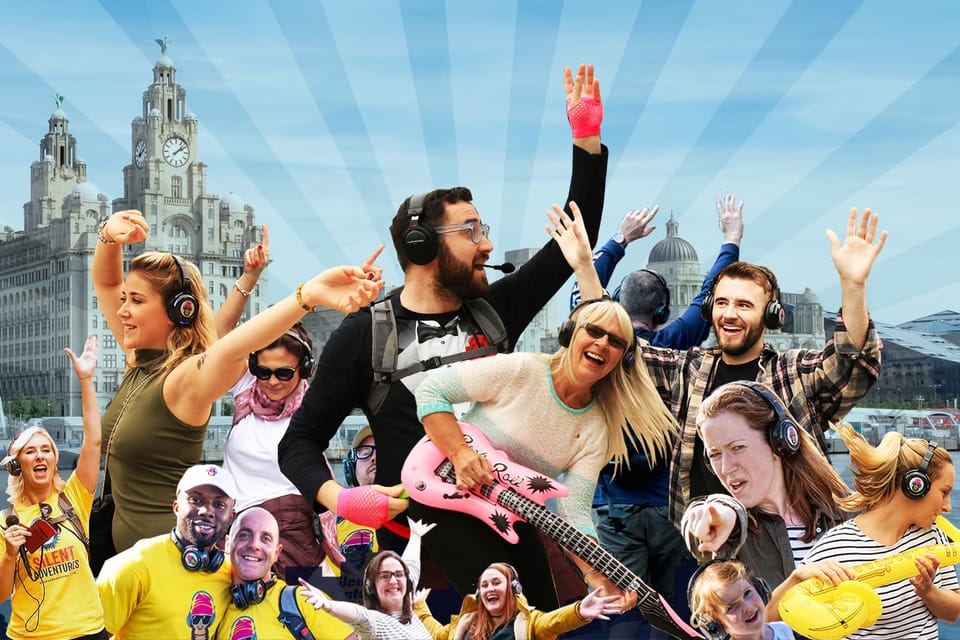This bustling scene captures a dynamic silent disco event beneath a vibrant blue, slightly cloudy sky adorned with streaming stripes. At ground level, a diverse crowd festively dances, with many participants donning yellow shirts emblazoned with "SILENT ADVENTURES." Among them is a blonde woman, energetically raising her left arm and brandishing a red object with her right hand. She, like many others, wears headphones, immersing herself in the music. Another notable detail is a person in a black shirt with a backpack and microphone, adding to the lively atmosphere. Dominating the upper left corner is an iconic clock tower, reminiscent of Big Ben, standing tall among other buildings in the background, enhancing the picturesque quality of this joyful gathering. The lower left foreground highlights a woman with an inflatable pink guitar, further emphasizing the festive, musical spirit of the event.